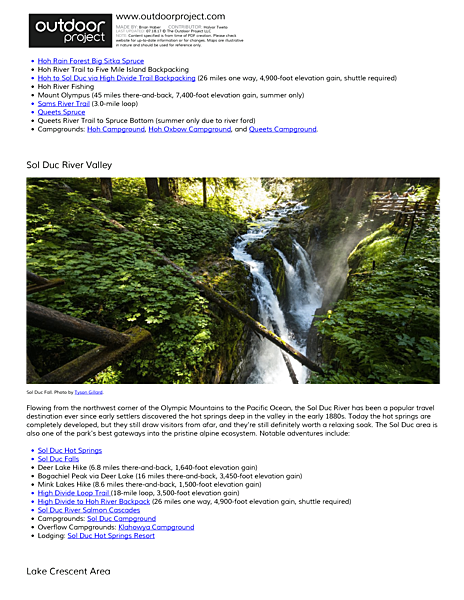The image features a detailed layout of an outdoor scene, as well as an informative text box in the top left corner. The top left-hand corner of the image contains a small black rectangle with the word "outdoor" written in bold white lowercase letters, followed by "project" in non-bold white lowercase letters. To the right of this, in black font, is the URL www.outdoorproject.com. Below this URL, some text is displayed in black and blue fonts, with the blue font text underlined, though it is difficult to decipher due to the small font size.

The central portion of the image showcases a horizontal rectangular photograph of a tranquil river winding through a dense forest. The river is bordered by numerous tree trunks and lush green grass, creating a serene natural scene. A section of the river forms a small waterfall, adding an element of dynamic beauty to the picture.

Below the image, a descriptive caption provides additional context: "Flowing from the northwest corner of the Olympic Mountains to the Pacific Ocean, the Sol Duc River has been a popular travel destination ever since early settlers discovered the hot springs deep in the valley in the early 1880s. Today, the hot springs are completely developed, but they still draw visitors from afar and are well worth the relaxing soak. The Sol Duc area is also one of the park's best getaways into the pristine alpine ecosystem. Notable adventures include Sol Duc Hot Springs, Sol Duc Falls, and Deer Lake Hike (6.8 miles there and back), among other attractions."

This detailed caption not only highlights the stunning natural beauty captured in the photograph but also provides historical context and lists popular activities in the Sol Duc area.